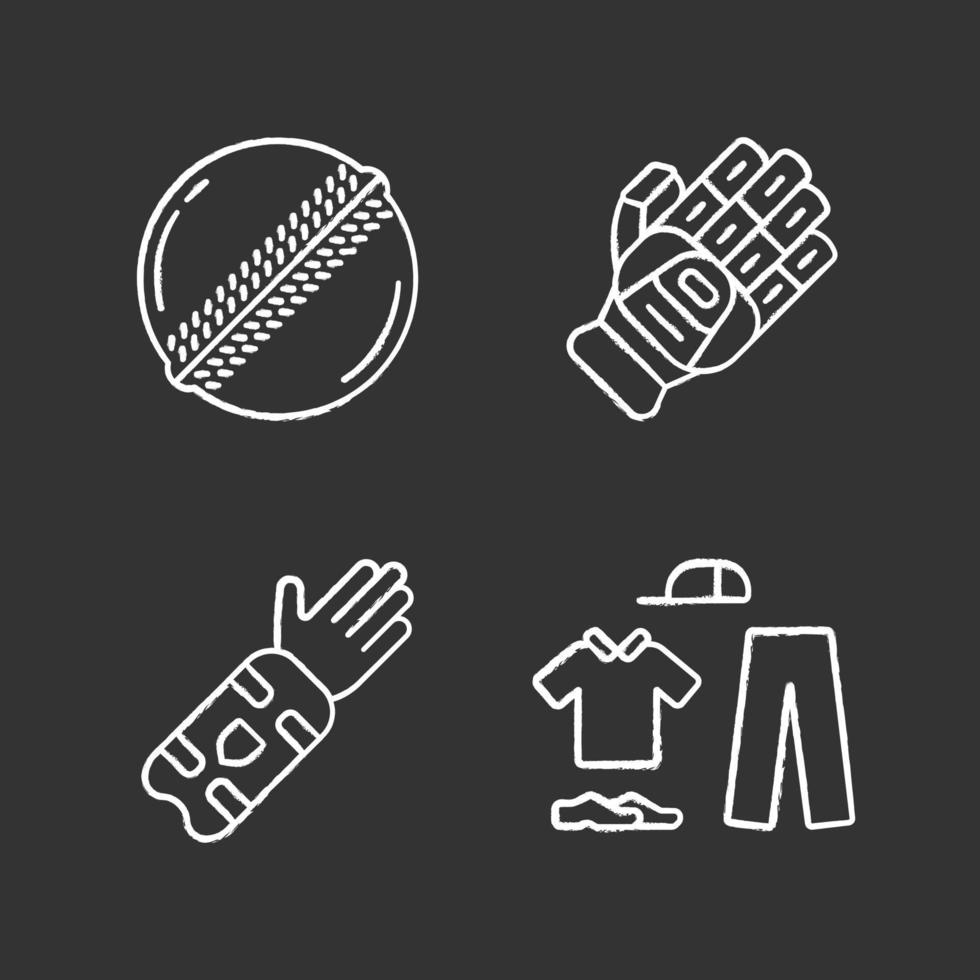This is a detailed black and white image with a pure black background and white, computer-animated style drawings divided into four quadrants. In the upper left quadrant, there's a round ball, possibly a stylized or shiny sphere with a ridge running through the center and two lines of small decorative spots along the ridge, indicating light reflections. The upper right quadrant features a glove or hand, depicted with squared-off fingers and thumb, each joint marked by a white line, and the back of the hand marked with a curved design. The bottom left quadrant shows a simplified hand in a gauntlet, with the gauntlet appearing larger and wider than the hand, featuring curved lines along its sides and a pointed design in the middle. Lastly, the bottom right quadrant portrays a simplified outfit, consisting of a hat, a collared T-shirt, pants, and shoes, all outlined in thick, bold white lines against the black background.